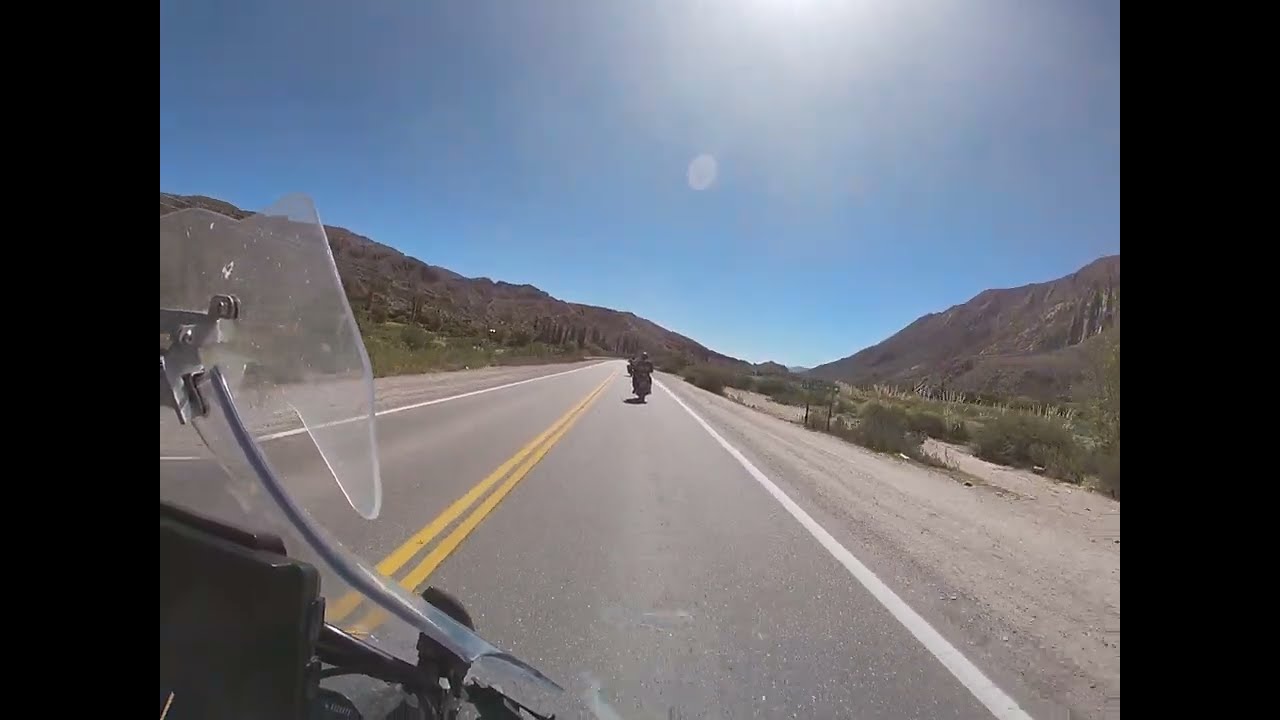This image, taken from the first-person perspective of a motorcyclist, captures a scenic ride through an arid, mountainous landscape. The photograph, which has thick vertical black borders giving it a square appearance, shows a clear, blue sky with the sun visible at the top center, creating a slight glare and blur that suggests it was taken through a transparent motorcycle windscreen. In the foreground on the left, part of the motorcycle's handlebar and insect guard are visible. The road is a two-lane highway with double yellow lines down the middle and white lines marking the shoulders. Ahead, two fellow motorcyclists can be seen, both wearing black helmets and outfits. The surrounding terrain is marked by dry, brown mountains with patches of grass and low shrubbery. The bright, sunny conditions and lack of visible clouds underscore the arid nature of the landscape.